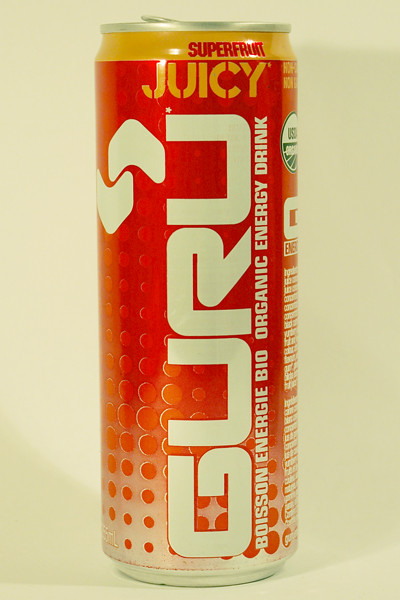In the foreground, a prominent aluminum can stands upright. The can’s logo, predominantly red with accents of orange and gold, captures immediate attention. The top of the can features a band of rich gold, and the word "Superfruit" is emblazoned in uppercase red and black letters beneath it. Juxtaposed below, the word "JUICY" is horizontally printed, with distinctive vertical slashes through some letters and a diagonal slash through the 'Y,' revealing the can’s background color.

The striking letters "GURU" run vertically down the can in white, with most corners rounded except for a few angled ones, reminiscent of the NASA worm logo's geometric aesthetic. Below "GURU," the inscription "Bison Energy Bio Organic Energy Drink" appears in all caps and white, creating a subtitle effect. 

The intricate backdrop of the can features gradients transitioning from white to various shades of red, dotted with contrasting circles that blend into the design. The pattern appears textured with a mix of light shades and black shading, giving a slight tan effect under specific lighting conditions.

In the far background, barely discernible, are nutritional facts and additional information, creating a sense of mystery. The overall aura of the image is modern and edgy, with stark contrasts and a sophisticated interplay of colors and shapes.